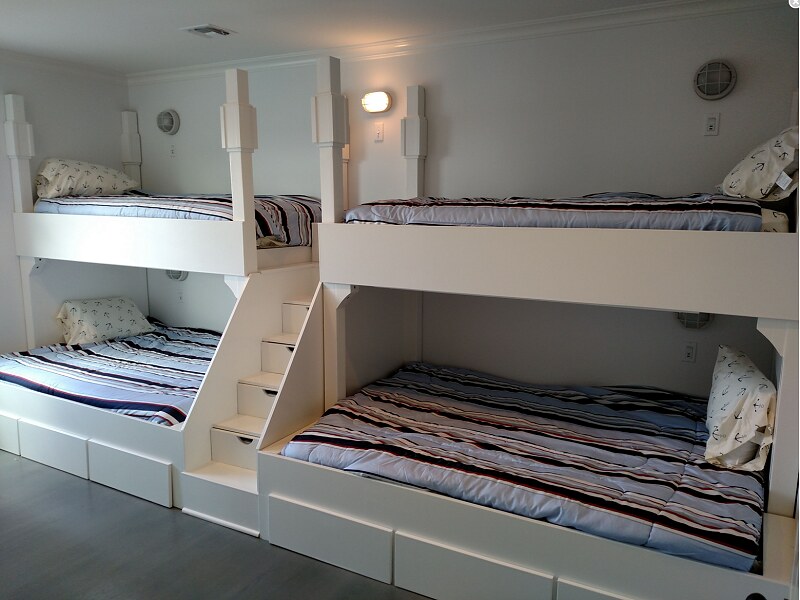The image depicts a well-organized bedroom with a unique bunk bed configuration. The room features two sets of bunk beds, each part of a single, elaborately designed white wooden frame. Positioned beside each other, the bunk beds are separated and connected by a central staircase with five steps, which also serves as a storage unit with drawers. The lower bunks appear to be full-size beds, while the upper bunks are twin-size. The beds are adorned with blue, black, and white striped bedding, and each comes with a white pillow showcasing an anchor pattern. The floor is a dark hardwood, complementing the gray walls. Mounted on the walls, each bunk bed has its own individual lamp, with one centrally located light currently switched on. The ceiling is light gray with a small section visible, featuring a ceiling vent. Overall, the room combines functionality with aesthetics, offering ample storage and a cohesive color scheme.